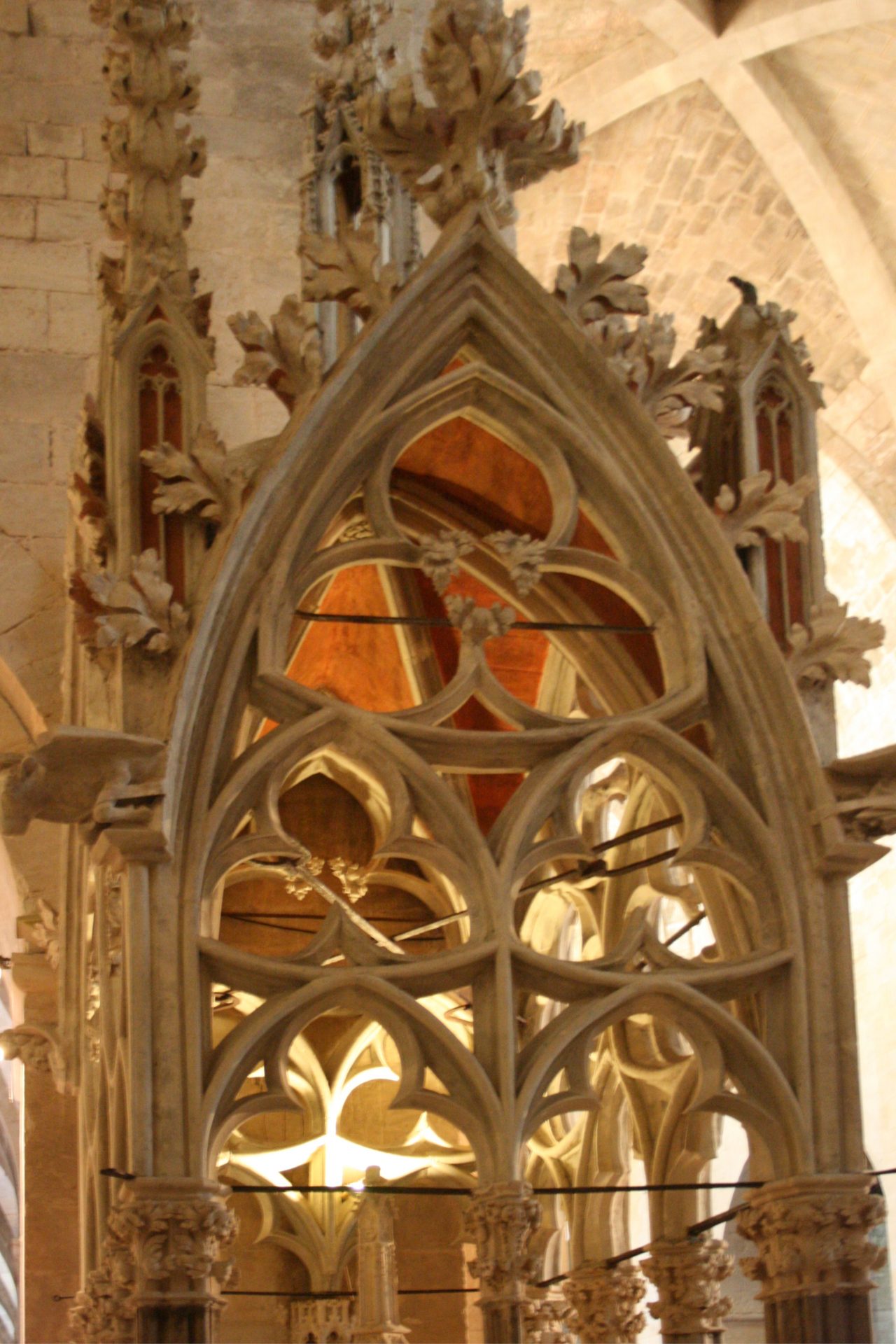This photograph captures a meticulously crafted triangular stone archway, likely an ancient architectural element dating back several centuries. The archway, suggestive of a historical church or place of worship, is adorned with a series of intricate three-petaled floral embellishments. There are five such decorations: one prominent one crowning the top of the arch, followed by two smaller ones directly beneath it, and another set of two lower down. The archway is framed against a backdrop of elaborate stone carvings, featuring intricate leaf motifs that add to the overall grandeur. This beautifully detailed stonework appears to be housed within a domed structure composed of both stone and brick, underscoring the rich heritage and craftsmanship of the period.